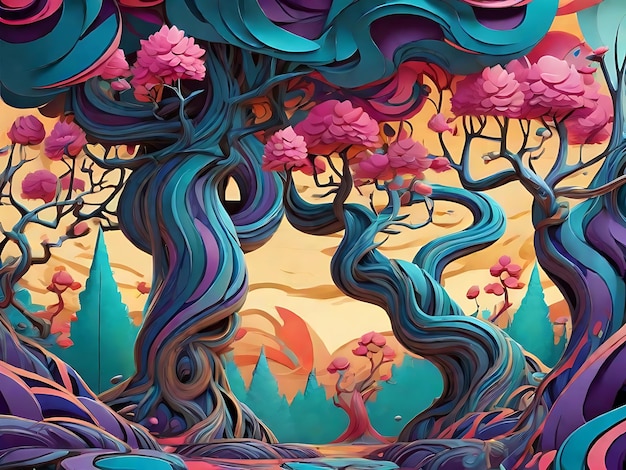The image is an abstract, artistic depiction of a whimsical forest, characterized by its wavy, almost hair-like tree trunks in hues of blue, teal, and purple. These trunks spiral and curve around themselves, giving a fantastical, psychedelic feel to the scene. The forest floor is adorned with vibrant pink, purple, and pink hues, creating an otherworldly, almost water-like appearance. Some trees stretch toward a distant horizon, exhibiting silhouettes of green, pine-like forms. The foliage varies in texture: while some branches blossom with cherry blossom pinks that share the trunks' wavy quality, others feature pink blooms resembling bird feathers or potato chips. The sky is a striking yellow and orange gradient, suggesting the time might be either sunset or sunrise, although the sun remains unseen. This vivid and imaginative portrayal, filled with an array of colors, is both whimsical and distinctly abstract, creating an entrancing, dream-like forest landscape.